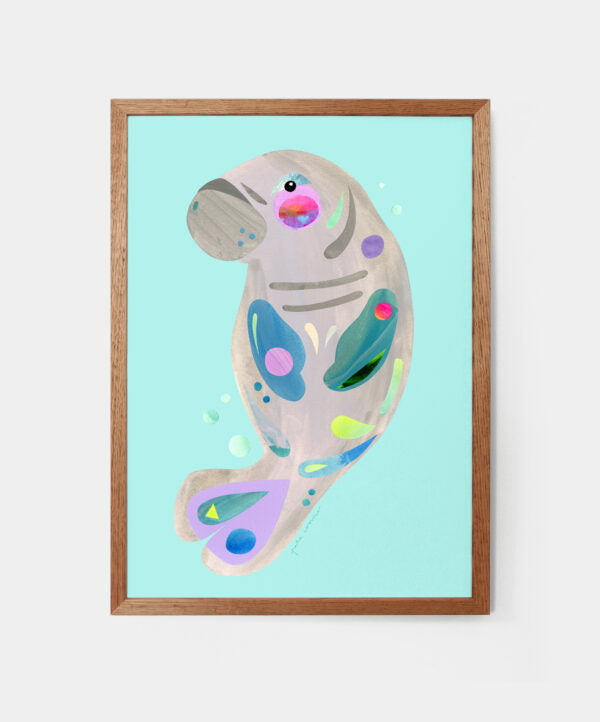This image depicts a whimsical painting of a manatee, framed in a medium to dark brown wooden frame set against a white wall. The background of the painting is a light teal, almost aqua color. The manatee is primarily gray with an array of vibrant hues adorning its form. Its head is oriented towards the left-hand side, and its fins curl inward. The body features a mix of abstract patterns with colors like pink, purple, green, and blue. Notable details include a purple heart on its tail, multi-colored spots and splashes along its back and flippers, and a splotch of pink and purple on its cheek resembling a blush. The intricately patterned flippers display different colors and shapes, such as a green flipper with a reddish-pink spot and a blue flipper with a purple spot. The eye is dark, accentuated with a light blue above and pink below, featuring a circle with hot pink on top and light purple on the bottom and a blue heart incorporated. The manatee’s belly and tail are visible, enhancing the impression that it is floating serenely in water.